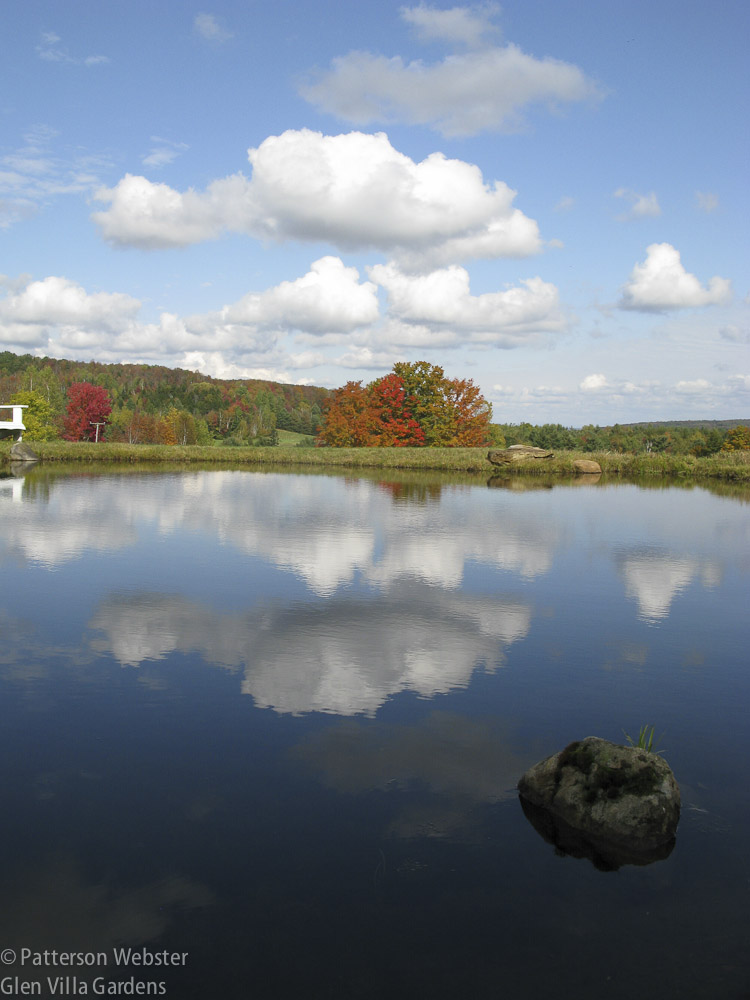This photograph captures a serene lake scene, bordered by a lush, wooded area displaying the vibrant colors of early fall. The far side of the lake boasts a mix of green, red, and orange foliage, indicating the changing seasons. Above, the sky is a canvas of large, white, wispy clouds set against a sunny blue backdrop, all of which are perfectly mirrored in the lake's calm waters, creating a stunning, albeit slightly blurred, reflection. In the bottom right corner, a small dark gray rock adorned with delicate green vegetation protrudes from the water. Just off the left edge of the photograph, a camper or small hut is barely visible, suggesting minimal human presence in this tranquil setting. The photo also bears a copyright notice in white lettering on the bottom left, reading "Patterson-Webster, Glen Villa Gardens," adding a final touch to this beautifully captured moment in nature.